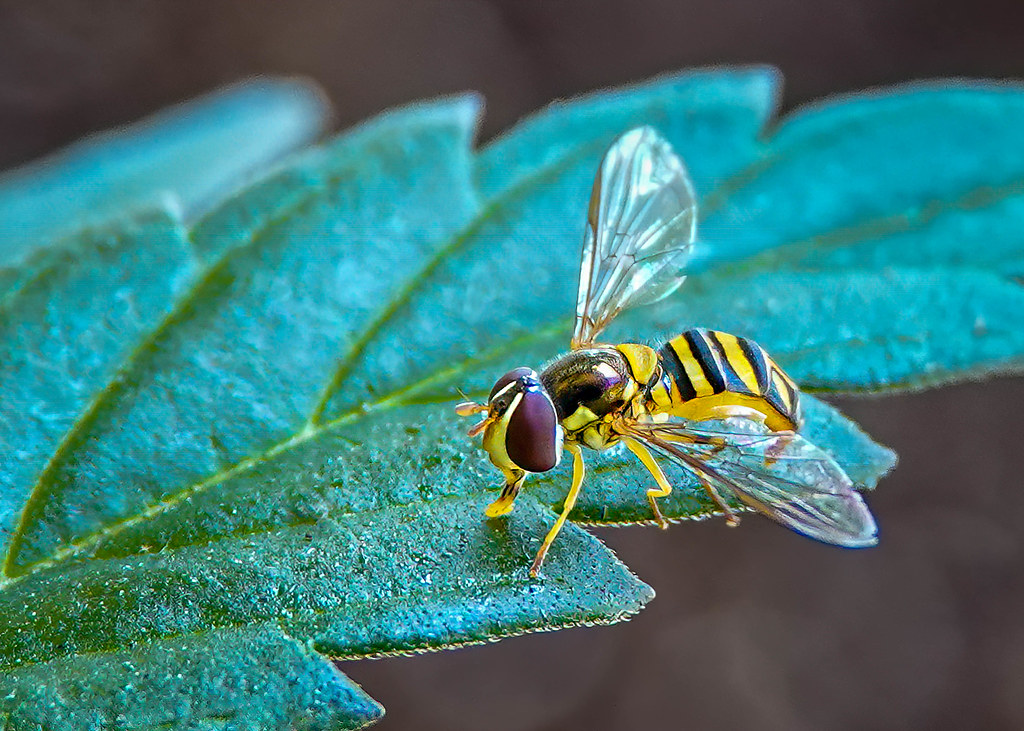This captivating nature photograph showcases an ultra-close-up view of a vibrant green leaf glistening with moisture, possibly from recent rain, displaying its intricate veins and seven distinct pointed tips. Centrally positioned, a bumblebee with vivid yellow and black stripes on its abdomen is captured in exquisite detail. The bee's two large, dark brown eyes dominate its head above its delicate yellow legs and prominent antennae. One of the bee’s two see-through wings is splayed to the side while the other stands straight up. The insect, appearing to explore the edge of the leaf, seems engaged in searching for pollen or nutrients, providing a striking glimpse into its natural behavior.